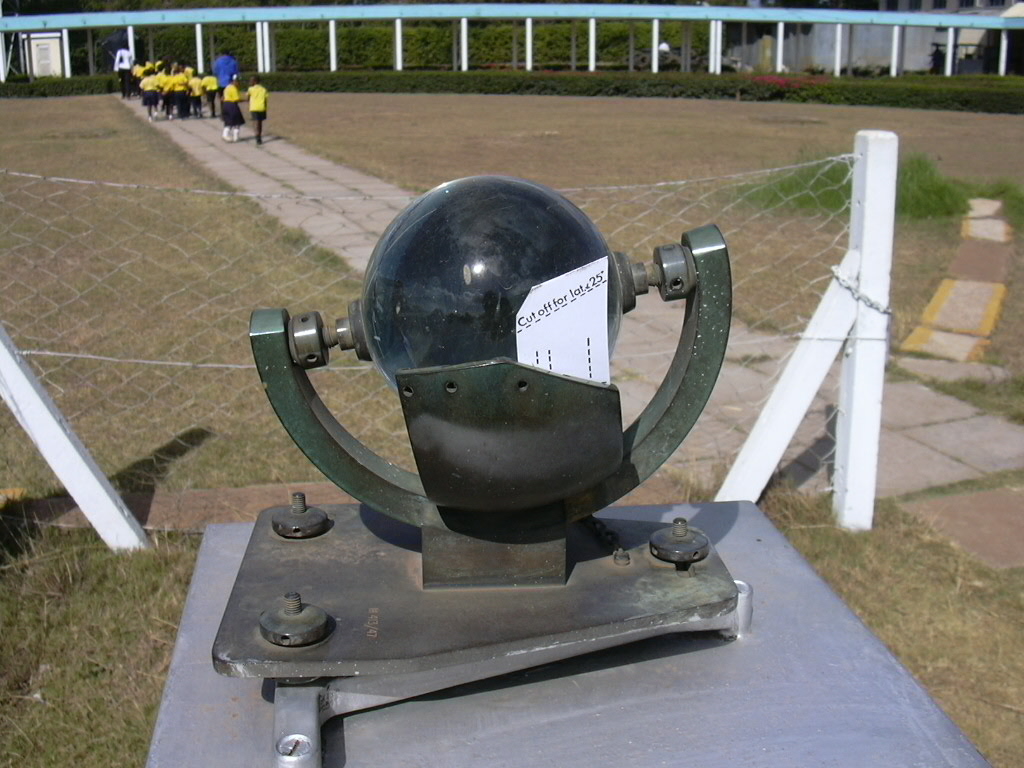This photograph showcases a complex mechanism, likely an astronomical or solar measurement instrument. The centerpiece of the image is a sturdy metallic structure made from steel and iron, featuring a spherical object mounted on a half-crescent support. The instrument bears a tag with partially readable text, mentioning "cut off for late," though the rest is obscured.

The scene is set in what appears to be a school environment. In the background, a group of children dressed in yellow and black uniforms are seen walking across a field in the top left quadrant of the image. They are accompanied by two adults, one wearing blue and the other in white. The children and adults are moving away from the camera's perspective, traversing a field enclosed by a net that separates them from the foreground.

The mechanism itself is elevated on a platform several feet above the ground, suggesting its importance or the need for precision in its placement. The overall setting and the detailed composition of this photograph provide a glimpse into an educational or scientific context, perhaps used to teach or demonstrate principles related to astronomy or solar measurements.